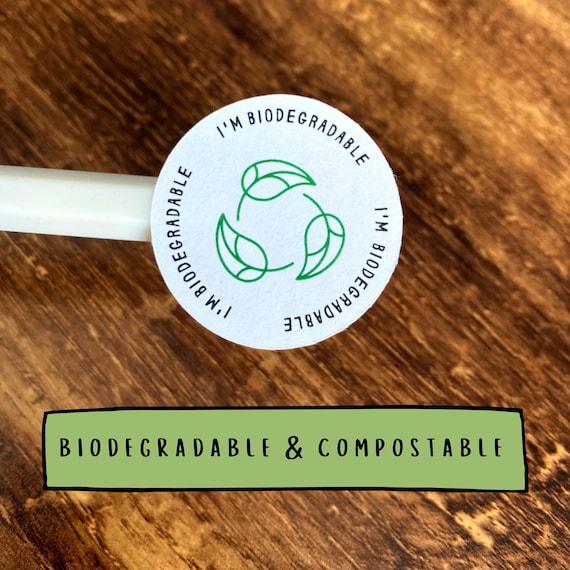The image displays a white circular sticker placed in the middle of a white tube emerging from the left side. The sticker features a central logo composed of three green leaves arranged in a circular pattern, represented in line art. Encircling the logo, black text spirals around, reading "I AM BIODEGRADABLE" in all caps. Below the sticker, a green rectangular label with a black border contains the text "BIODEGRADABLE AND COMPOSTABLE" in bold black capital letters. The background consists of a brown hardwood surface with diagonal grains extending from the top left corner to the bottom right, showcasing a gradient from lighter to darker tones in various areas.